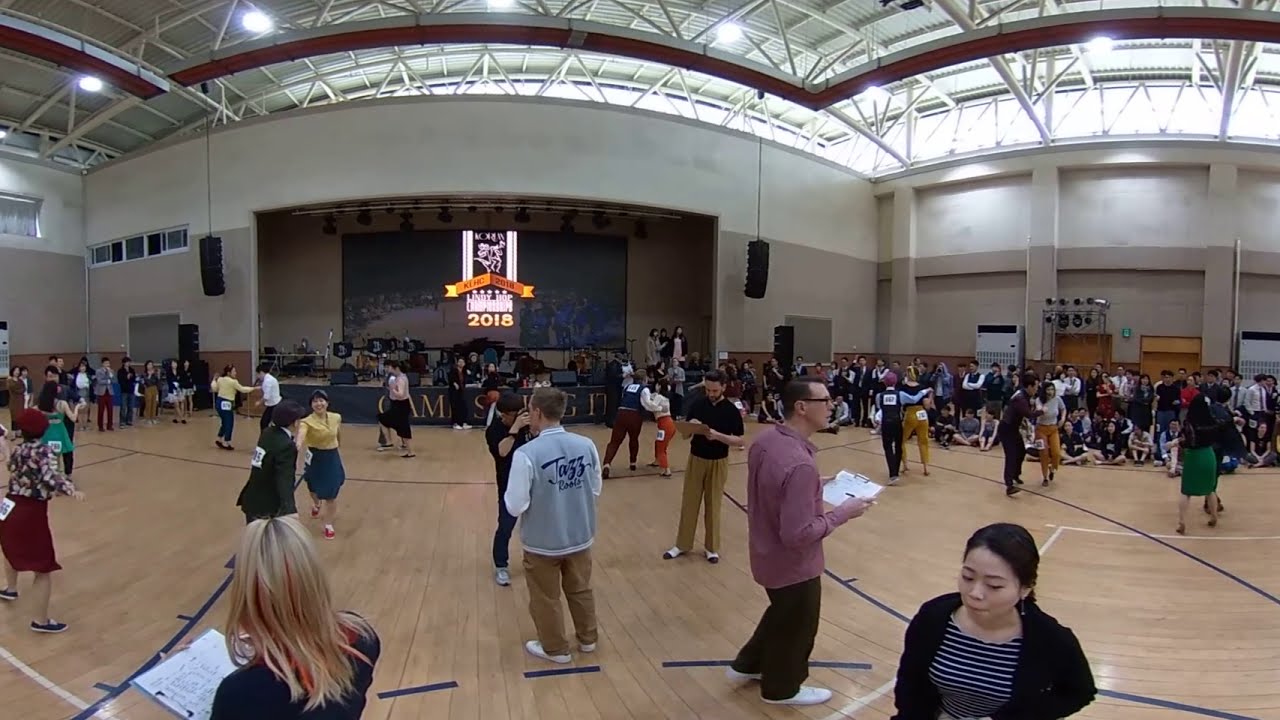The photograph captures the vibrant scene of a large indoor gymnasium with distinct features and a bustling crowd. The spacious gym is adorned with white metal beams and red ductwork on the ceiling, illuminated by bright ceiling lights, creating a lively atmosphere. The gym's walls transition from dark brown at the bottom to light grey at the top, enclosing a wooden basketball court marked with tape for various sports activities.

In the center of the gym, numerous people, possibly participants in a dance competition, fill the space. Many of them wear white numbers on their backs, indicating they are dance contestants. Several couples, comprising males and females, are positioned across the floor as if in the midst of performing intricate dance routines. A notable figure stands out in the middle, a man wearing a grey vest with the word "jazz" inscribed in cursive, suggesting a jazz dance-off or marathon.

Lining the gym’s perimeter, spectators—likely students—watch intently. Some individuals hold boards with notes, possibly judging the dancers. On the back wall, a large stage features a monitor displaying the year 2018 in gold font alongside a black school emblem with a white border. The stage, though equipped with musical instruments, remains unoccupied, emphasizing the event's focus on the dance competition. Overall, the gymnasium is a well-lit, dynamic setting hosting a lively and engaging dance event.